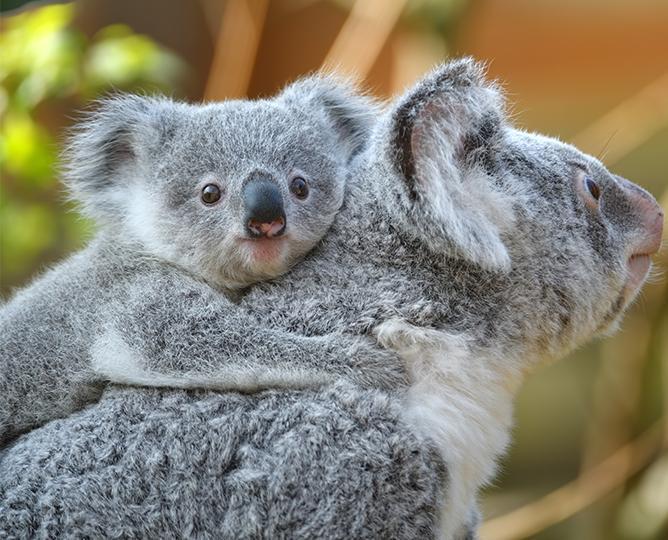In this photograph, two koala bears, likely a mother and her child, are the central focus. The adult koala is positioned in the center, facing to the right, revealing a profile that includes her gray fur, a white chest, and one prominent ear with white inner fur. Clinging to her back, the smaller koala looks directly at the camera with its head tilted forward, displaying both of its ears, eyes, and a large black nose. The background is artistically blurred, combining tones of green, brown, and tan, suggesting a natural habitat with indistinct foliage and branches. The upper left side of the background is highlighted by vivid green hues, while the right side features duller green shades, adding to the depth and ambiance of the natural setting.